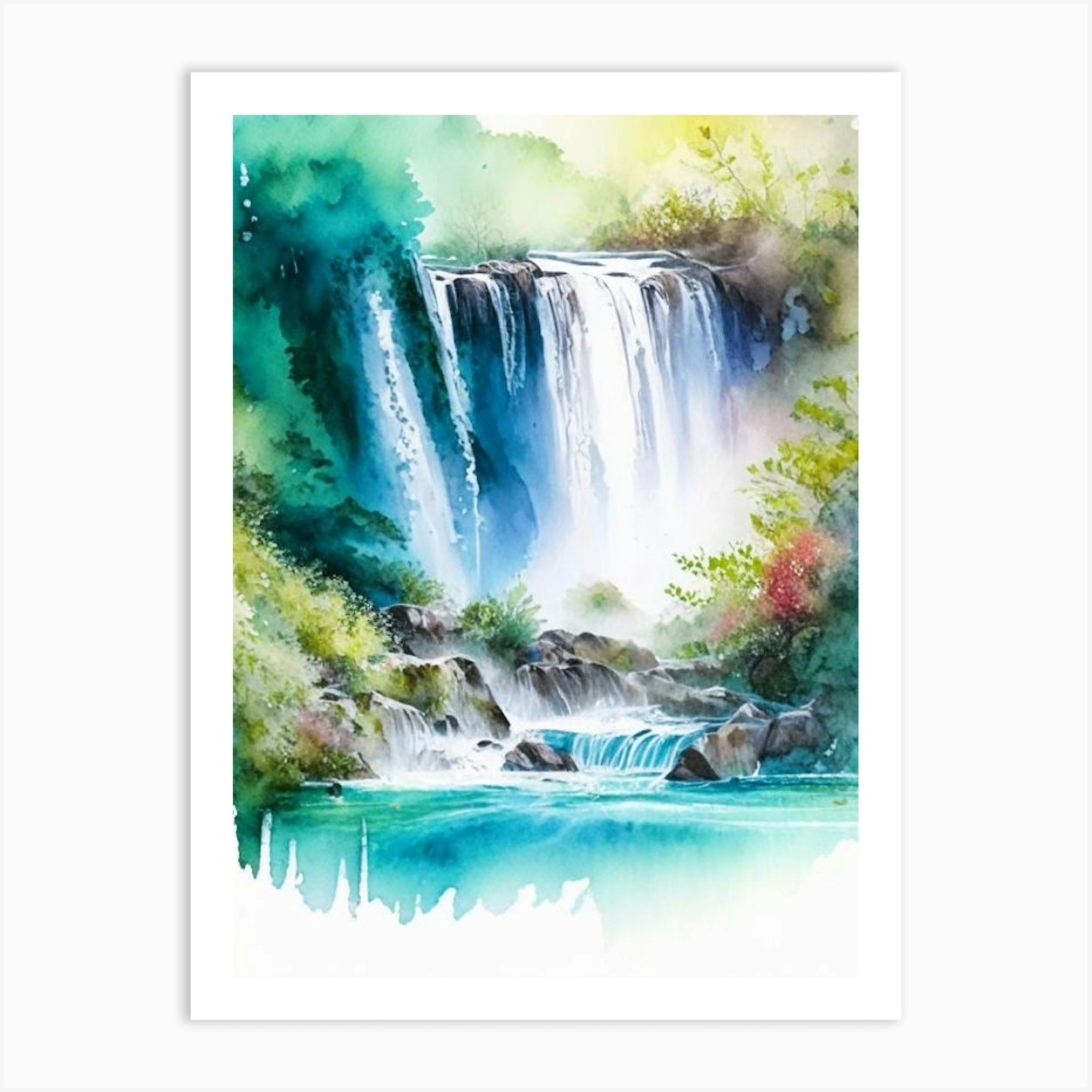The image is a watercolor painting of a natural waterfall, depicted on a white portrait canvas with a white frame. The painting features a majestic waterfall cascading from the top, with white and blue water flowing gracefully. The scene includes lush greenery with grass and flowers at the top, and sprigs of greenery surrounding the waterfall. A pink and white flower is prominently visible on the right side. The water becomes crystal blue as it flows over gray rocks adorned with moss, creating smaller cascades before pooling into a serene turquoise lake at the bottom. Clouds and blue spray add a dynamic touch to the upper part of the painting. The painting contains shades of blue and various greens, blending seamlessly to create a tranquil and picturesque natural scene.